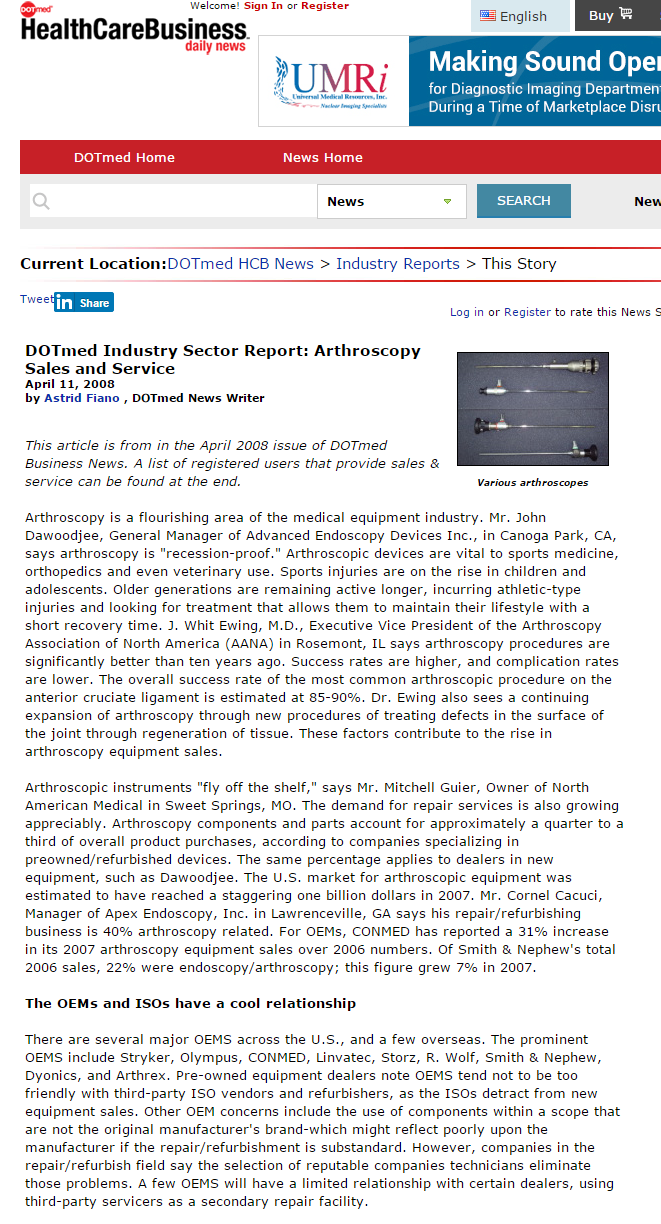**Caption:**

The image highlights the importance of signing up and registering for diagnostic imaging services, especially during times of microphone disruption. The "Dot Med Hall" and "News Hall" serve as critical areas for staying updated with the latest healthcare visit news and advancements in diagnostic imaging, as exemplified in the April 2018 issue of Dot Med Business News. This issue features a noteworthy article on the cathroscopy of cells, providing a detailed analysis and industry sector report on its significant growth, with an 11 to the 7th rate observed by Astro Japan. The article also includes a comprehensive list of registered users integral to the supply chain.

Astroscopy, a burgeoning field within the medical community, is spotlighted. Mr. John Dawoodji, General Manager of Advanced Endoscopy Devices in Kanagawa Park, California, applauds the technological advancements in astroscopy and emphasizes its value to their partners. It is noted that OEMs (Original Equipment Manufacturers) and ISOs (Independent Service Organizations) have a strong correlation in cell imaging across the United States. Prominent OEMs in this sector, mentioned in the image, include Stryker and Pompeo Scala, although there is a caution against committing to a specific OEM at this stage. 

This detailed caption underscores the complexity and collaborative nature of advancements in diagnostic imaging and astroscopy within the medical industry.